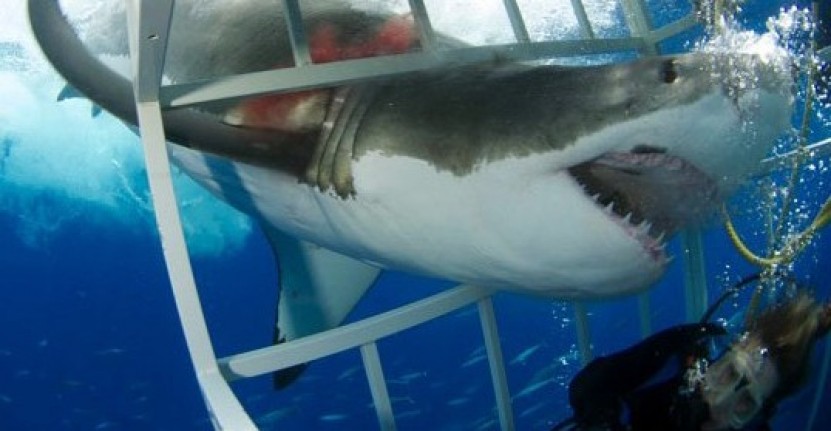In this vividly detailed underwater photograph, a great white shark is depicted in the act of aggressively breaching a shark cage, creating a dramatic focal point. The shark has forced its head through a horizontal opening in the cage, its powerful body still outside, as it attempts to reach the diver within. The great white's mouth is open, showcasing its daunting array of sharp teeth, perilously close to the diver who is partially visible in the bottom right corner, with their brown hair, goggles, and air supply equipment connected by numerous hoses. The ocean water is a deep, dark blue, and blood is visible near the shark's gill, indicating injury likely caused by its frantic efforts to penetrate the cage. The image is a color photograph, capturing the realism and tense atmosphere of the underwater encounter against the stark backdrop of the vast ocean.